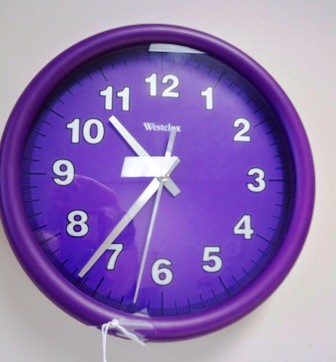This close-up color photograph captures a vividly detailed view of a round wall clock, set against a light gray backdrop. The clock stands out with its striking bright purple hue, featuring an outer rim with a metallic sheen and a clock face in a slightly different shade of purple. The analog clock face is marked with white numerals, making it easy to read the time. The brand name, barely legible, is positioned just below the number 12, beginning with a possible 'W.' The clock's minute, hour, and sweep second hands are also white, creating a sharp contrast against the purple face. The time displayed on the clock is approximately 10:38, or 22 minutes until 11.